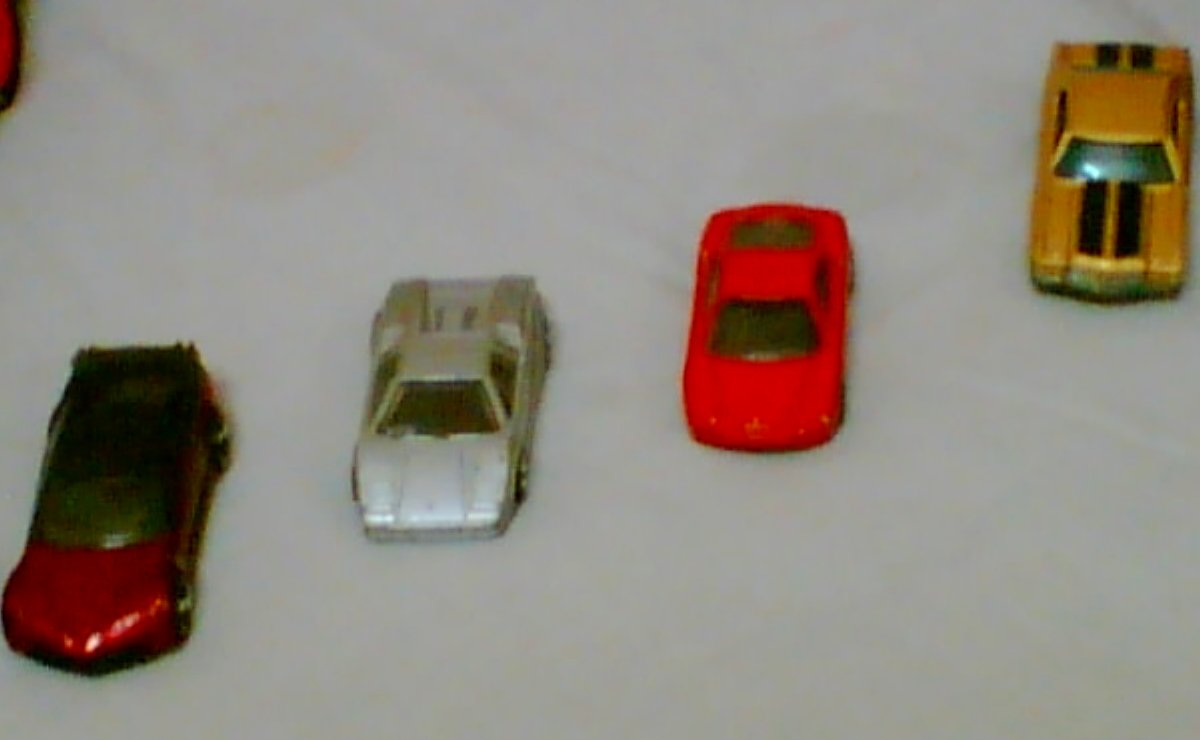A photograph captures four small toy cars, reminiscent of Matchbox or Hot Wheels, aligned diagonally on a white surface, potentially vinyl with some yellowish stains. Despite the image's blurriness and low quality, details of the cars are discernible. Starting from the bottom left, the first car is a dark red or maroon sports car with a black top. Next to it is a silver, boxy car with black wheels, embodying an 80s DeLorean style. The third car is bright red with black-tinted windows, featuring a modern, rounded sports car appearance. The fourth car, in the top right, is yellow with two prominent black stripes running from front to back, resembling a 70s or 80s muscle car. The cars' windows are darkly tinted, and the overall image includes a slight glimpse of an additional object in the upper left, potentially part of another toy.